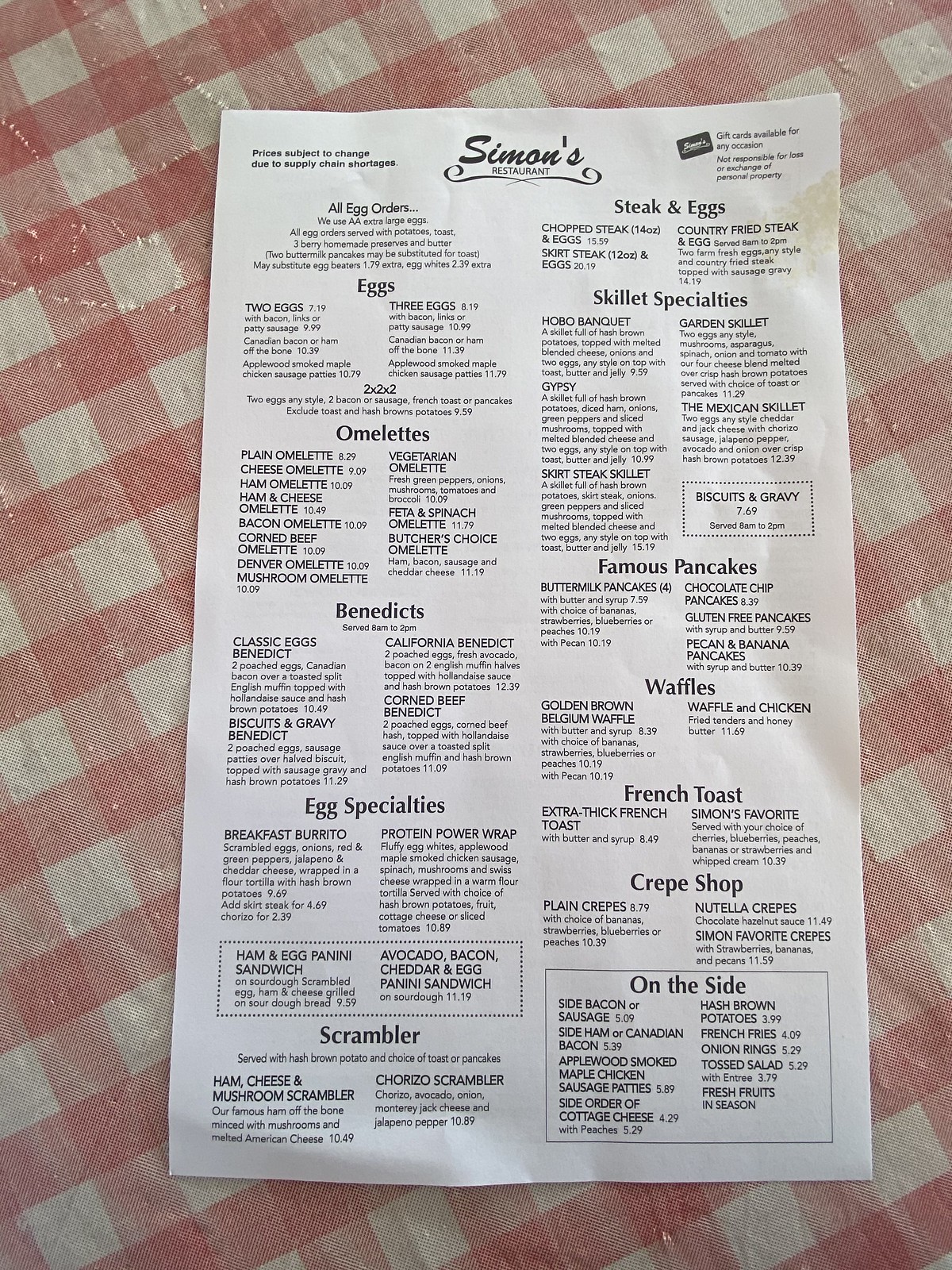The image showcases a detailed menu resting on a red gingham print tablecloth. The menu, which resembles a legal size sheet, is white with black text and is organized into a long, narrow format. At the top, the name "Simons" is elegantly scripted in cursive, followed by the word "restaurant" in plain text and a decorative scroll line beneath it.

The menu is divided into two main columns:

- **Left Column:**
  - It begins with the heading "All Egg Orders," providing a brief description.
  - Subsequent sections with larger font headings include:
    - Eggs
    - Omelets
    - Benedicts
    - Egg Specials
    - Scrambler
  - Each of these categories lists various options and their prices in smaller font underneath.

- **Right Column:**
  - Headings in this column include:
    - Steak and Eggs
    - Skillet Specialties
    - Famous Pancakes
    - Waffles
    - French Toast
    - Crepe Shop
  - At the bottom right, enclosed in a black-outlined box, is the heading "On the Side."
  - Each section provides a detailed list of offerings and their respective prices in smaller font.

The overall aesthetic of the menu suggests a classic, homey dining experience, enhanced by the red gingham tablecloth backdrop.